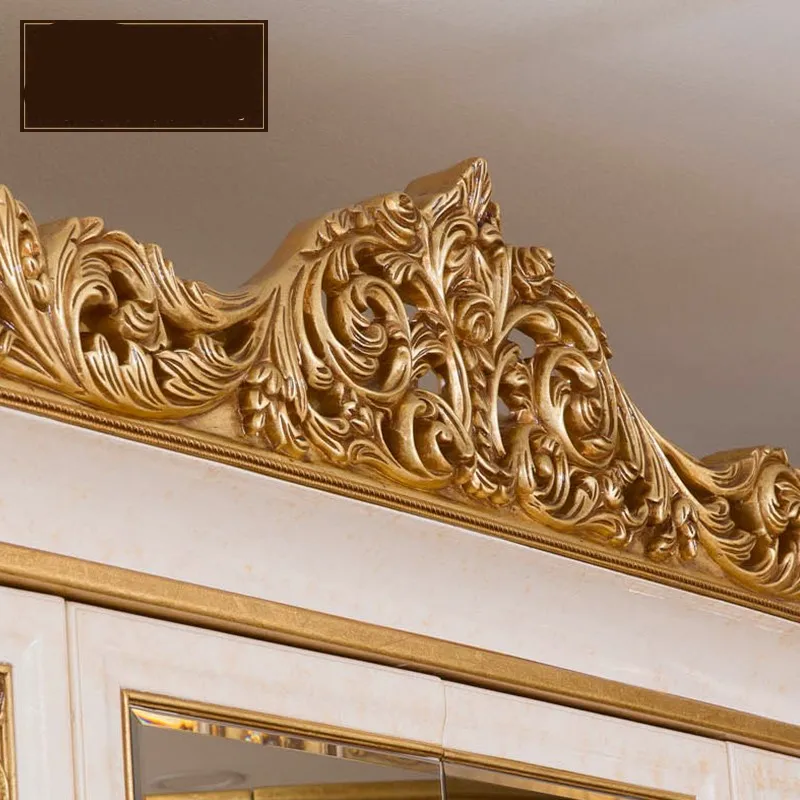The photograph depicts the upper portion of a meticulously maintained, ornate Victorian-style mirror or vanity. The frame showcases an elaborate gold design that features intricate looping and floral patterns, gracefully complemented by white outlining. The gold appears meticulously painted onto the white frame, which forms a harmonious border that runs horizontally across the image. At the top left corner, a brown rectangular box is visible, possibly part of the frame's detailing or an adjacent object. The background consists of plain white walls, emphasizing the cleanliness and well-preserved state of the mirror. The surface of the mirror is flawless, free from scratches, and meticulously maintained, with no visible text to detract from its vintage elegance.